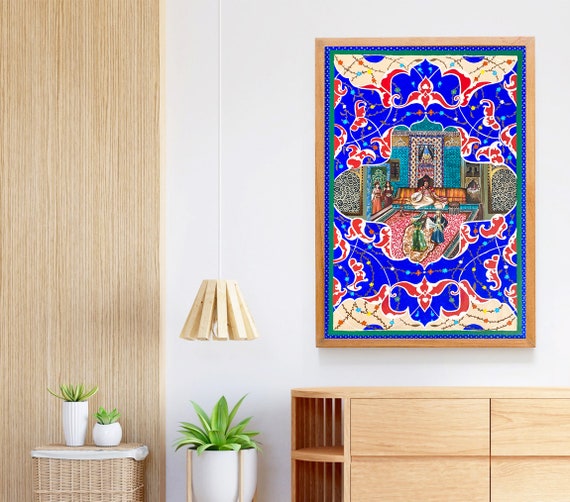In this photograph of a living room, the composition highlights a vibrant, colorful painting as its focal point. The painting, set in a natural tan frame, showcases an ornate, royal scene with a bright blue background, and intricate designs in reds and whites. The centerpiece of the artwork depicts a regal figure seated on a couch, flanked by women in long dresses and other figures in old-fashioned, ornate clothing, against a red carpet and blue squiggle designs. This artwork hangs on a white wall above a tan chest of drawers that matches the warmth of the wood elements throughout the room.

To the left of the dresser, a wicker basket or hamper with a lining inside can be seen, topped with two small potted plants—one in a vertical vase, the other in a lower vase. A larger potted plant in a white ceramic pot with a tan holder stands beside the smaller plants. Above this arrangement, a light fixture dangles from the ceiling, casting a warm glow. The leftmost part of the scene shows a wood-panel wall, integrating the tan and natural wood tones that complement the contemporary pine-style furniture staged within the room.